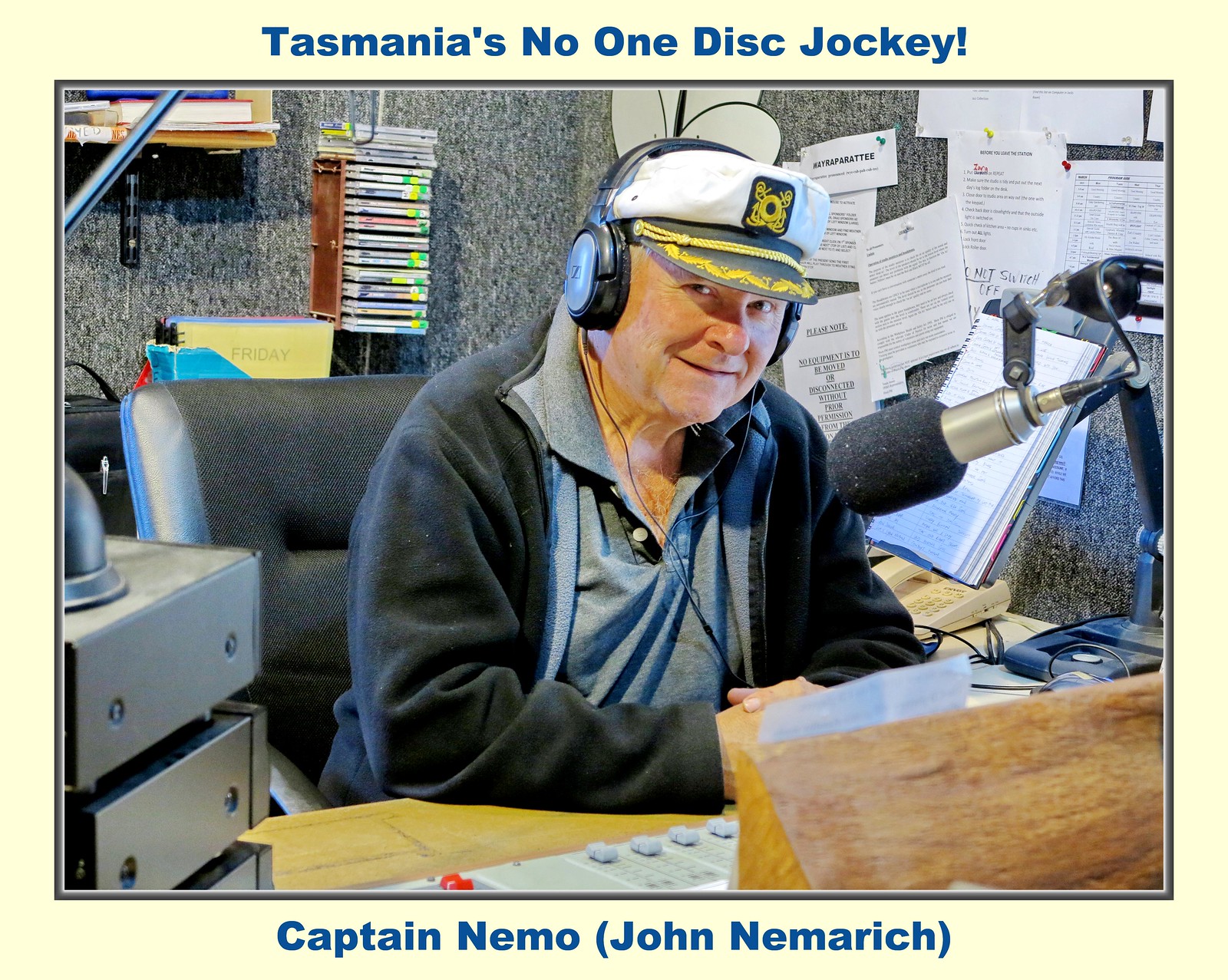The image is a horizontal-rectangular photograph set against a light yellow background that frames the picture. At the top of the image, blue text reads "Tasmania's No. 1 Disc Jockey!" while the bottom features the caption "Captain Nemo (John Nemerich)" also in blue.

The photograph depicts an older gentleman, presumably Captain Nemo, seated at a radio station control panel. He is wearing a distinctive white nautical captain's hat with a black brim adorned with gold designs, reminiscent of the skipper's hat from "Gilligan's Island." He is also donning a blue jacket over a light blue shirt and has earphones with a "Z" on them.

Captain Nemo sits in a black chair, leaning slightly towards a large microphone mounted on a stand that extends from the desk. His hands are clasped in front of him, and he is smiling subtly at the camera. In front of him, the control panel is equipped with sliders, and various broadcasting equipment surrounds him. Behind him, a bulletin board is cluttered with pinned papers and a stack of compact discs is visible, with additional notes and CDs organized against a gray and white wall. To his upper left, a shelf holds what appears to be a book, adding to the busy and professional atmosphere of the radio station.

This detailed scene encapsulates Captain Nemo in the midst of his role as Tasmania's foremost disc jockey.